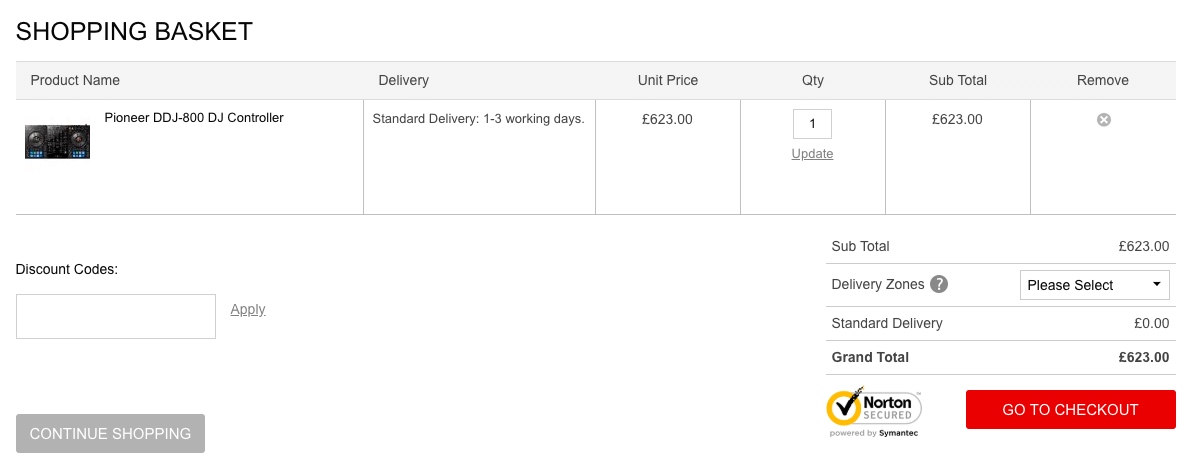The image depicts a detailed shopping basket interface on an e-commerce website, likely for purchasing electronic goods. At the top of the section, a "Shopping Basket" title is prominently displayed. Below it is a gray banner with columns labeled: "Product Name," "Delivery Dates," "Unit Price," "Quantity," "Subtotal," and "Remove."

In the main part of the basket, there is a listed product: a Pioneer DDJ-800 DJ controller. The delivery method for this item is "Standard Delivery (1 to 3 working days)." The unit price is shown as £623. The quantity is set to "1" in an editable box that allows for updates. An "Update" button is situated beneath this quantity box. The subtotal for the product is also £623. 

To the far right, there is a "Remove" option marked by a small "X" icon to delete the product from the basket.

Below the product information, there is a section titled "Discount Codes." Underneath, there is a text box for entering a discount code, flanked by an "Apply" link to the right.

To the right of the discount code section, a summary of the order is provided. This includes:
- Subtotal: £623
- Delivery Zones: A drop-down menu to select the delivery zone
- Standard Delivery: £0 (indicating free standard delivery)
- Grand Total: £623

At the bottom of the interface, there is a prominent red "Go to Checkout" button with "Go to Checkout" in bold white text.